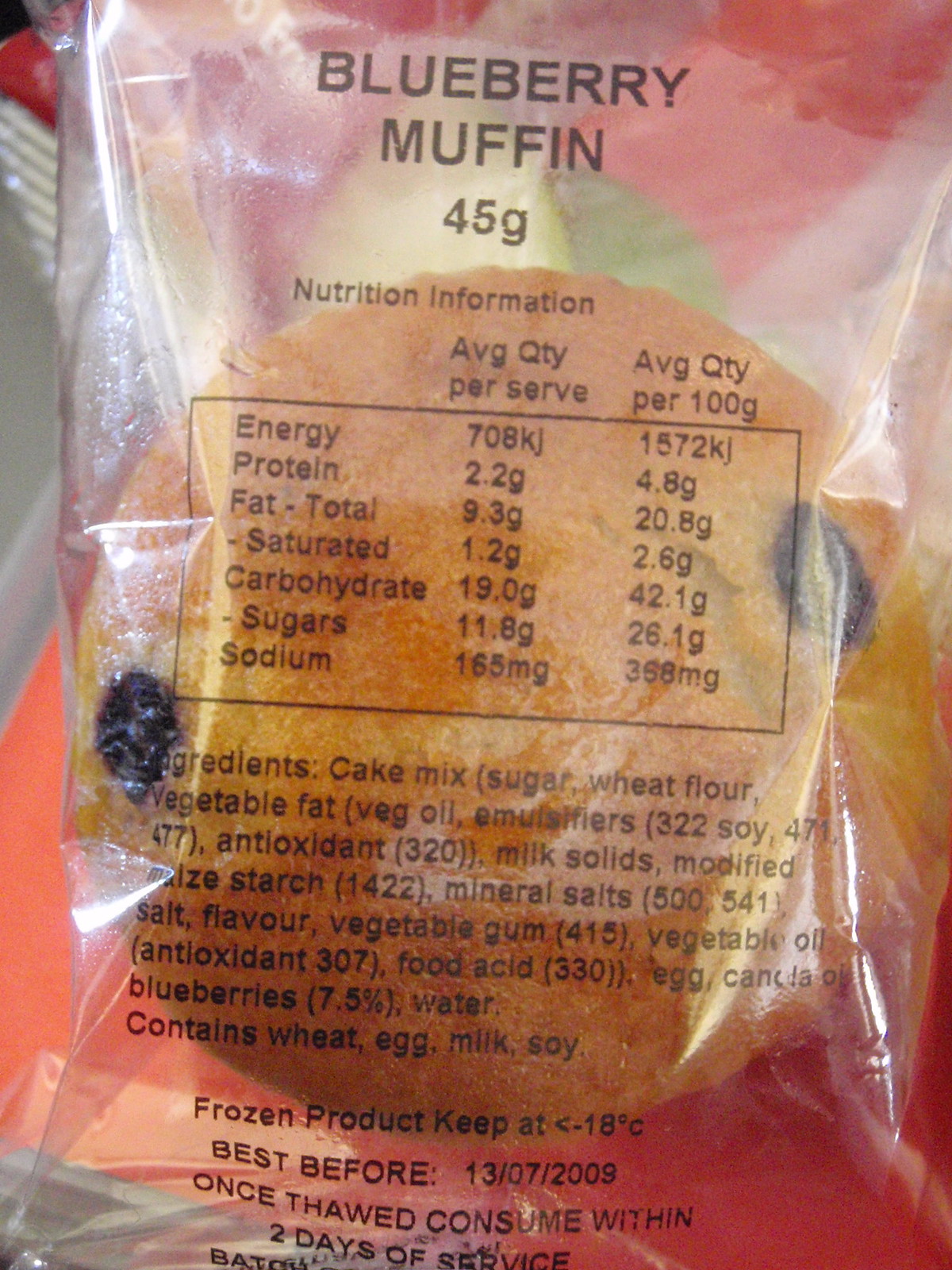In this image, a blueberry muffin is showcased, still enclosed in its clear plastic wrapper against a red background. The wrapper is printed with "Blueberry Muffin" in black, followed by the weight, "45G". Detailed nutrition information is displayed, listing average quantity per serving and per 100 grams: Energy (708kJ per serving, 1500/725kJ per 100g), Protein (2.2g/4.8g), Fat (total 9.3g/28.8g, saturated 1.2g/2.6g), Carbohydrate (19.0g/42.1g), Sugar (11.8g/26.1g), and Sodium (165mg/368mg). The ingredients include cake mix, sugar, wheat flour, vegetable fat, vegetable oil, emulsifiers (322, soy 471, 477), antioxidants (307, 320), milk solids, modified starch (1422), mineral salts (500, 541), salt, flavor, vegetable gum (415), egg, canola oil, and 7.5% blueberries. It contains wheat, egg, milk, soy, and is a frozen product to be stored below 18°C. The wrapper specifies "Best before 13-7-2009" and advises consuming the muffin within two days of thawing. The muffin itself is round and predominantly brown with visible dark bluish-purple blueberry dots.